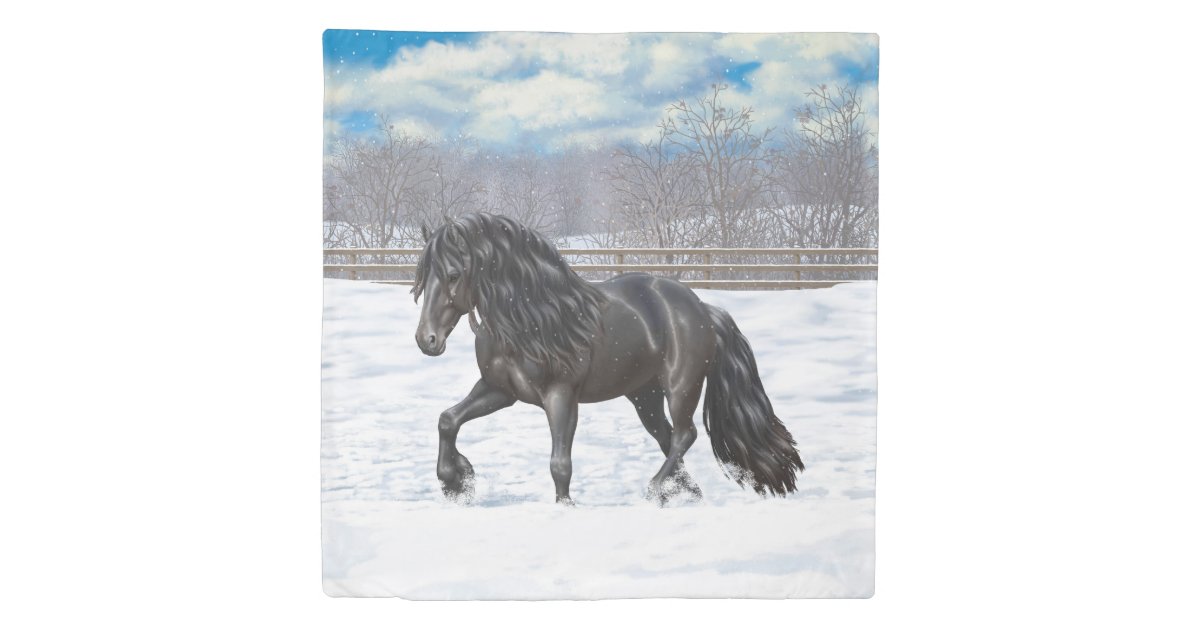The square illustration features a majestic black horse with a shiny coat, characterized by its long, dark mane and impressively bushy tail. The horse appears to be either skipping or running, sending snow flying into the air as it moves across a snowy landscape. The ground is deeply blanketed in snow, with snowfall contributing to the wintry scene. In the background, leafless trees and a three-post wooden fence add to the serene, frozen atmosphere. Beyond the fence and the trees, snow-covered hills stretch into the distance. Above it all, a blue sky, dotted with fluffy, cotton-like clouds and twinkling stars, completes the tranquil background.